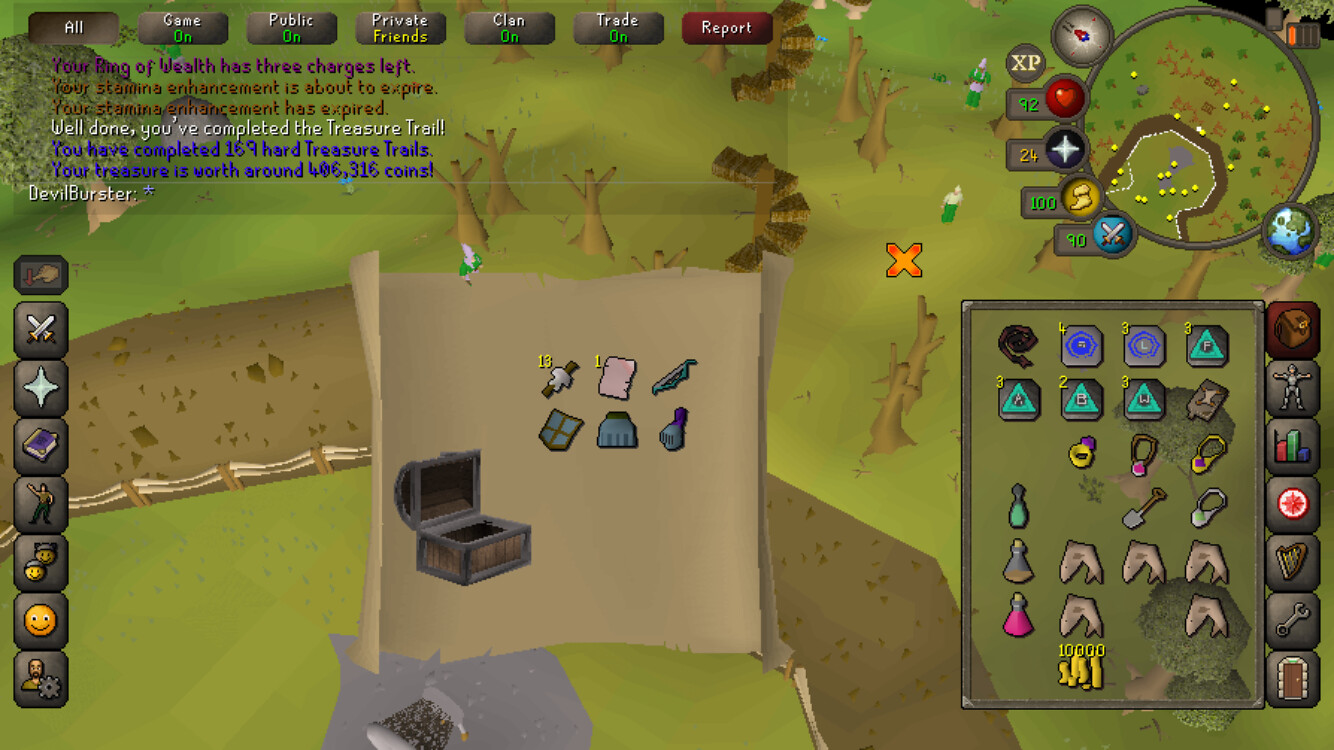In this image, which appears to be a video game screen set against a light lime green background, there is a central brown sheet of torn paper featuring a brown chest box. To the right of the chest are six pieces: four are gray, one is pink, and one white with brown, alongside the number 13, and a pink piece of white paper marked with the number 1. Additionally, on the right side, grayish items include a shovel and rings, with purple boxes displaying the numbers four, three, and three. A circular map outline is positioned at the top. On the left, dark gray buttons state "All," "Game On," "Public On," "Private Friends," "Clan On," "Trade On," and a red "Report" button with white lettering. Below these, there are gray boxes featuring a happy face, a star, two crossed swords, and a person. A brown trail extends downward, showing cut-off trees and an orange X. The scene is vibrant with pinks, greens, reds, browns, and yellows, suggesting a treasure hunt game with detailed elements and in-game notifications such as "your ring of wealth has three charges left," "your stamina enhancement is about to expire," "well done, you've completed the treasure trail," "you have completed 169 hard treasure trails," and "your treasure trail is worth 406,316 coins." The game's old-school graphics suggest it might be played on a computer rather than a modern console.